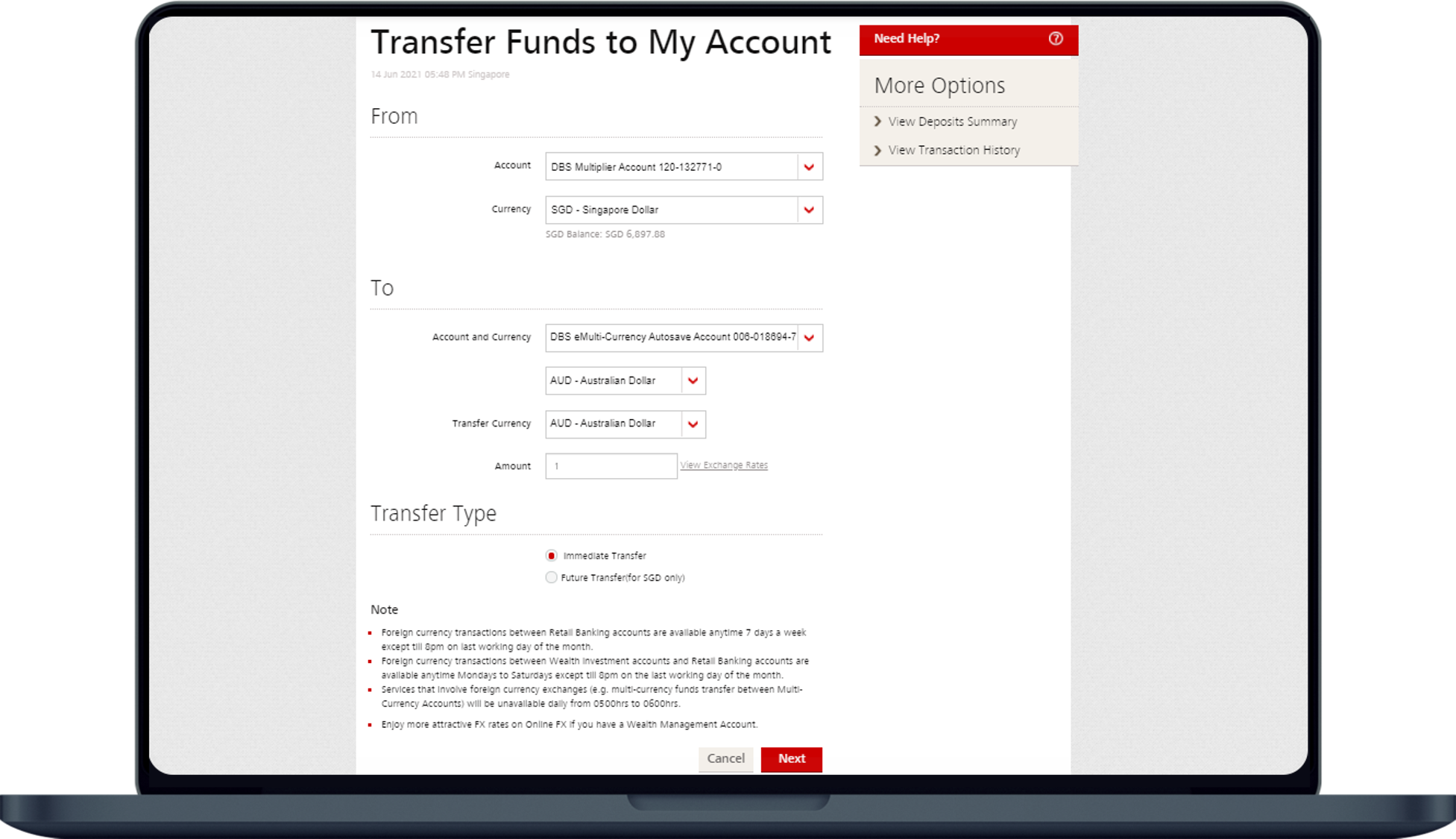In the image, a sleek MacBook is prominently displayed, its screen showcasing an online banking interface. The application appears to be processing a funds transfer. Specific text on the screen includes instructions and options such as "Transfer funds to my account," "I need help," "More options," "View deposit summary," and "View transaction history." The account information highlights a DBS Multiplier Account with the number 120-132771-0, holding a balance of 6897.88 Singapore Dollars (SGD). Additionally, there is information about a DBS e-multicurrency Autosave Account with the number 006-018694-7, designated in Australian Dollars (AUD). The user is preparing to transfer 1 AUD, specified as an immediate transfer.